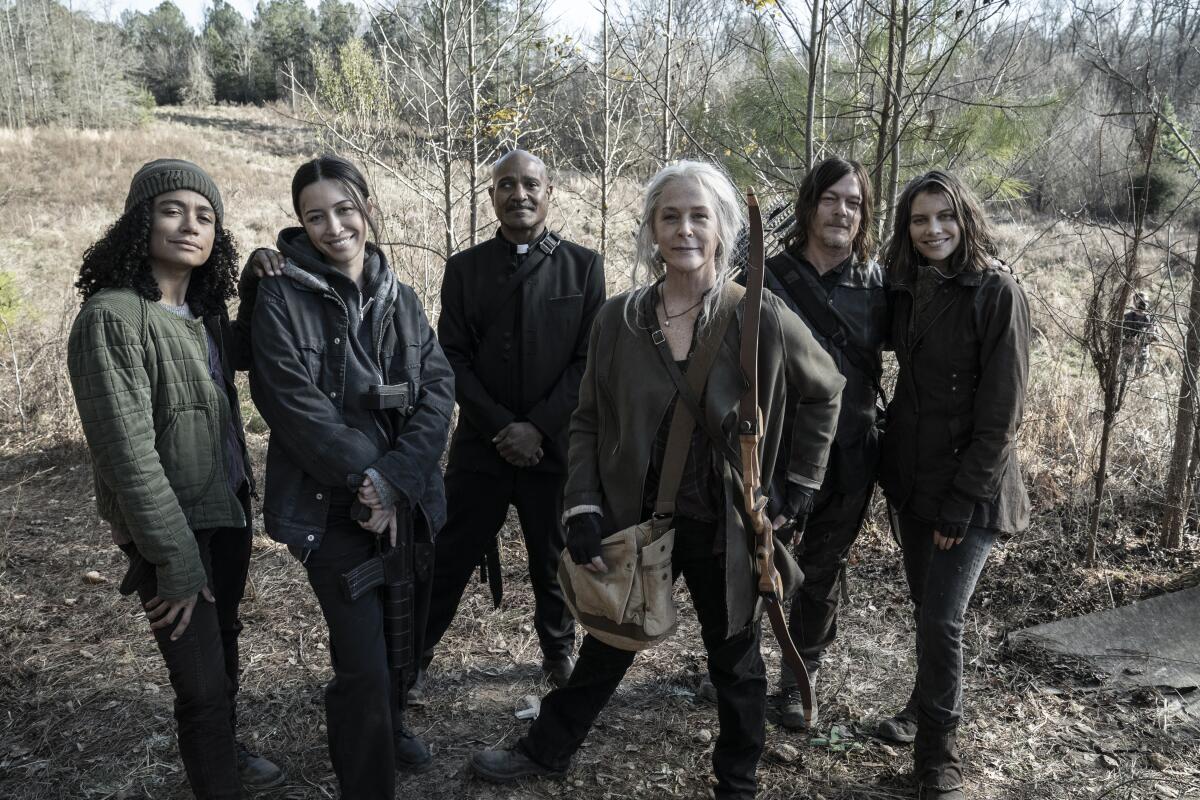The image depicts six cast members from "The Walking Dead" standing together in a forested, wintry setting. The cast members are all smiling at the camera. The group consists of four women and two men, each dressed in darker, mostly green and black attire, appropriate for the show's post-apocalyptic theme.

From left to right:
1. **First Woman:** Long curly hair, wearing an army-style jacket.
2. **Second Woman:** Wearing a darker green jacket with a purple shirt underneath, black pants, a gray beanie, and holding a gun in her criss-crossed hands.
3. **Third Woman (Front):** With gray hair, a blue jacket, a bag, and a bow and arrow.
4. **First Man (Back, Center):** African American, dressed as a priest with a black suit and a shaved head, holding a priestly demeanor.
5. **Fourth Woman (Middle Right):** Likely "Carol" (Melissa McBride), wearing a white hat and carrying a long machete with possibly a backpack.
6. **Second Man (Far Right):** Short hair, hinting that he might be Lauren Cohan's character, Maggie, wearing typical "The Walking Dead" survivor attire.

The background is a wilderness area with thin trees and grassy fields, accentuating the desolate environment. The lighting is grayish, aligning with the show's somber mood.